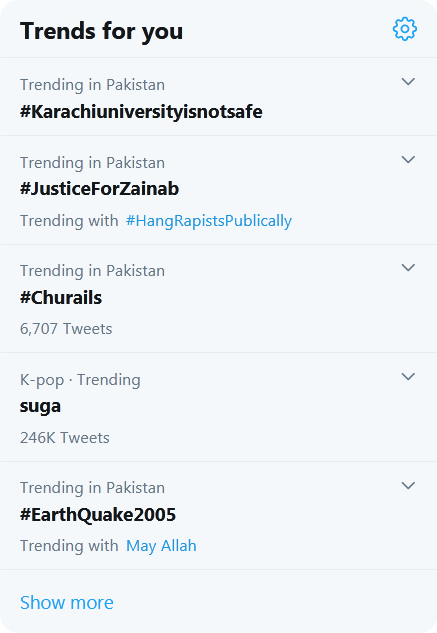Here is a more organized and detailed caption based on the provided information:

---

**Screenshot of Twitter Trending Topics**

The image showcases a gray rectangular section with black text, likely from a Twitter feed. At the top, it mentions "Trends for you" with a small blue gear icon. The trends listed include:

1. **Training Pakistan Karachi University** - This topic highlights safety issues at the Karachi University in Pakistan.
2. **Justice Resign on Trending with Hanging Rapists Publicly** - This trend discusses public demands for justice and resignations related to hanging rapists.
3. **Drop-down Training Pakistan True Rails** - A less clear trend with mentions of Pakistan and possibly railway training.
4. **K-pop Trending Sugar** - The popular Korean pop star, Suga, is trending with 246,000 tweets.
5. **Earthquake 2005 Trending with Me I'm Fine** - Refers to the 2005 earthquake, with users assuring "I'm fine" in their tweets.

Below the trends, there's an option labeled "Show more." This screenshot appears to be capturing current social media trends, specifically from Twitter, as it mentions tweet counts and topics.

---

This caption provides a clear and detailed description of the image while summarizing the key information from the original voice input.